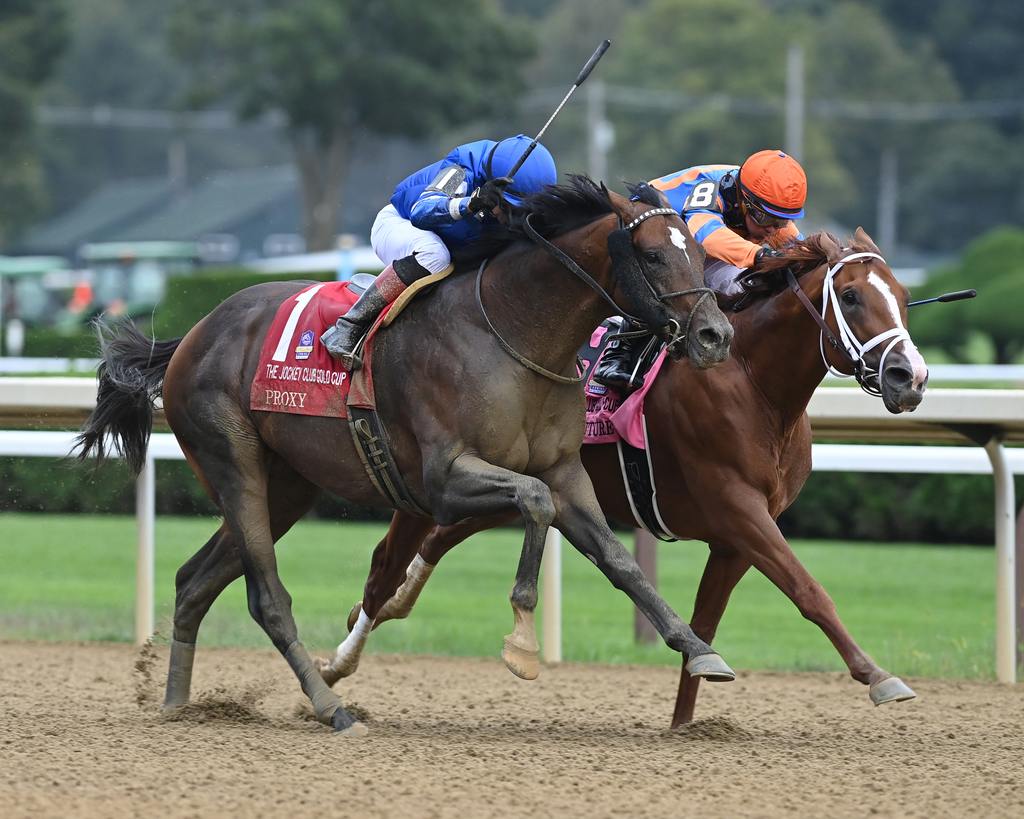This is a detailed image capturing the excitement of a horse race during daytime. The photograph focuses on two competitive brown horses running neck-and-neck on a dirt track. The leading horse is a slightly reddish-brown shade with a distinct stripe of white on its face, while the other, darker brown horse sports a smaller splash of white. Their jockeys are decked out in traditional uniforms; the jockey in the lead wears a blue and orange ensemble with the number eight displayed, paired with an orange and blue helmet. The jockey on the second horse is in a blue and white outfit with a corresponding white helmet. Both riders are equipped with riding sticks. Surrounding them, the track is encircled by a white barrier, beyond which lies a well-kept green grass field accented by trees and a couple of distant houses in the backdrop.